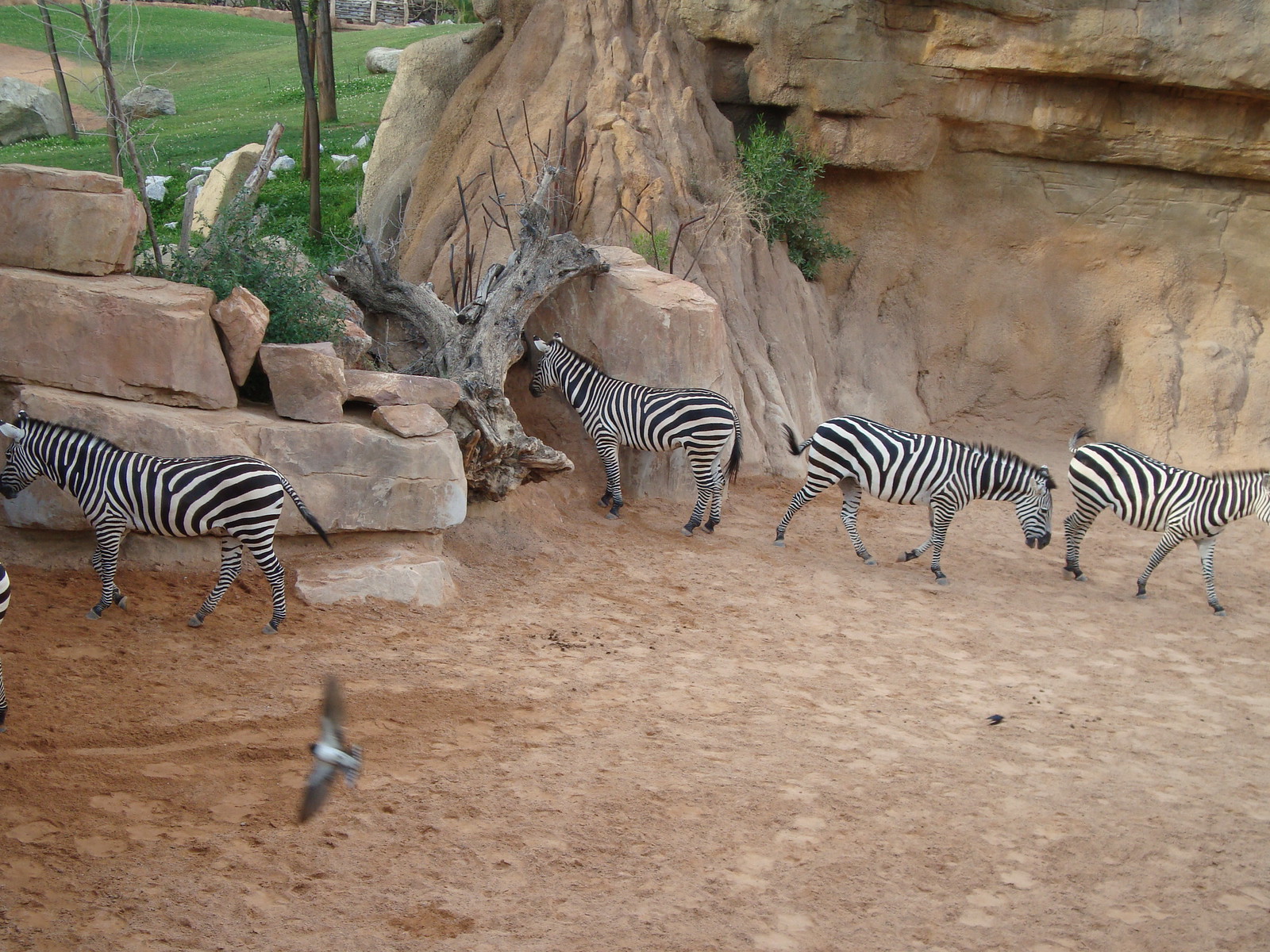This detailed color photograph captures a zoo exhibit featuring four zebras situated on a patchy light tan dirt ground. The zebras are distinct in their black and white striped patterns. Two zebras are positioned towards the right of the image, while the other two are facing left. The environment includes an artificial rock wall made up of stacked brown stones on both the left and right sides of the frame. At the center, a tree trunk adds a natural element to the enclosure. Surrounding the zebras and the rocky structures, there is green grass and thin, tall trees that enhance the exhibit's naturalistic appearance. A slightly blurry bird in mid-flight can be spotted near the bottom left of the image. In the distance, a fence is faintly visible, further emphasizing the zoo setting. There are no people or text in this traditional photograph.